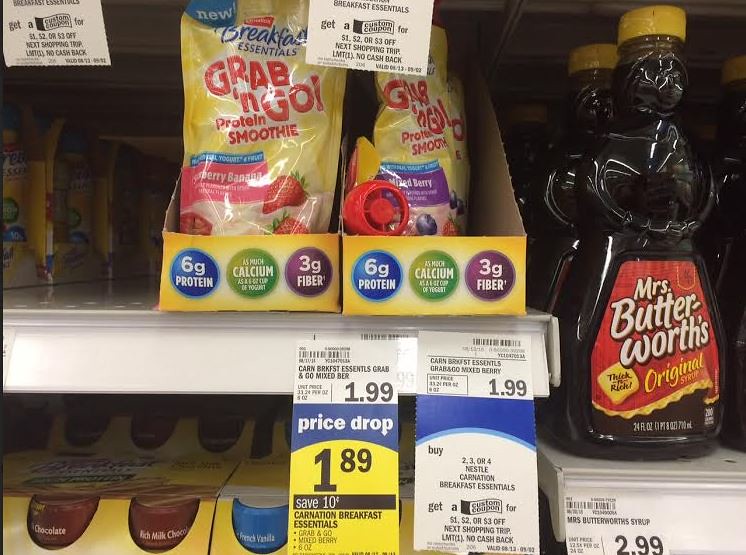The image depicts a grocery store aisle, focusing on three shelves stocked with products. The top shelf prominently features two bright yellow cardboard holders containing Carnation Breakfast Essentials Grab-and-Go Protein Smoothies. One holder has a Strawberry Banana flavor, illustrated with strawberries floating in a pool of white yogurt, and the other has a Mixed Berry flavor, showing blueberries and strawberries. Each holder boasts nutritional benefits: 6 grams of protein, as much calcium as a 6-ounce cup of yogurt, and 3 grams of fiber. The price tag for these items indicates a price drop from $1.99 to $1.89, with a special offer stating "Buy 2, 3, or 4 Nestle Carnation Breakfast Essentials, Get a custom coupon for $1, $2, or $3 off next shopping trip."

The second shelf below contains cans labeled “Rich Milk Chocolate,” though it is unclear if these are food items or a type of drink. 

The third shelf displays rows of Mrs. Butterworth's Original Pancake Syrup, each shaped like a woman with a yellow cap and labeled with a red apron adorned with yellow trim. The price tag beneath the syrup indicates a price of $2.99.